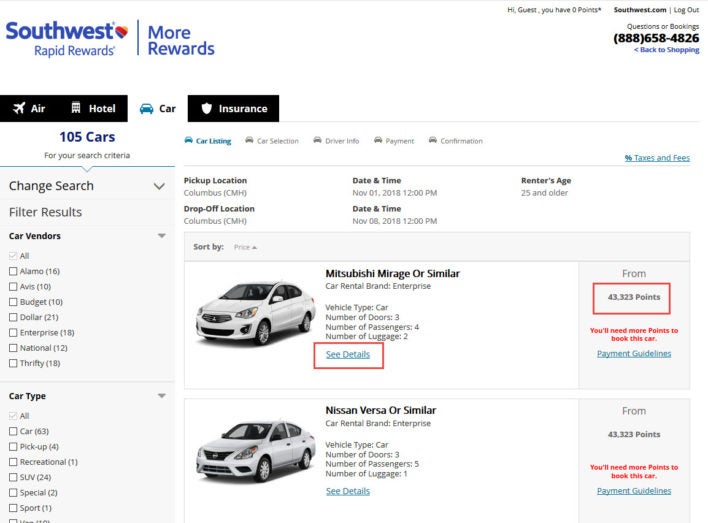Explore an extensive selection of rental cars tailored to your preferences with Rapid Rewards. Earn more rewards on air, hotel stays, and car insurance by calling 888-658-4826 or continue shopping for the perfect vehicle from our carefully curated options. We have 105 cars matching your search criteria; you can easily change your search parameters or filter the results by car vendors and specific attributes.

Highlighted deals include a Nissan Versa or similar compact car available for 3,328 points; this efficient silver car is perfect for city driving. Alternatively, consider a Mitsubishi Mirage or a similar vehicle for 3,823 points; depicted with a red box around the offer, this option stands out for its affordability. Both deals include detailed information about taxes and fees.

Conveniently select your pickup and drop-off location in Columbia, and specify your desired date, time, and renter's age. For added peace of mind, there's a shield icon next to the insurance option, ensuring you have all the necessary coverage. Start your journey with confidence and reward yourself with prime choices and exceptional service.